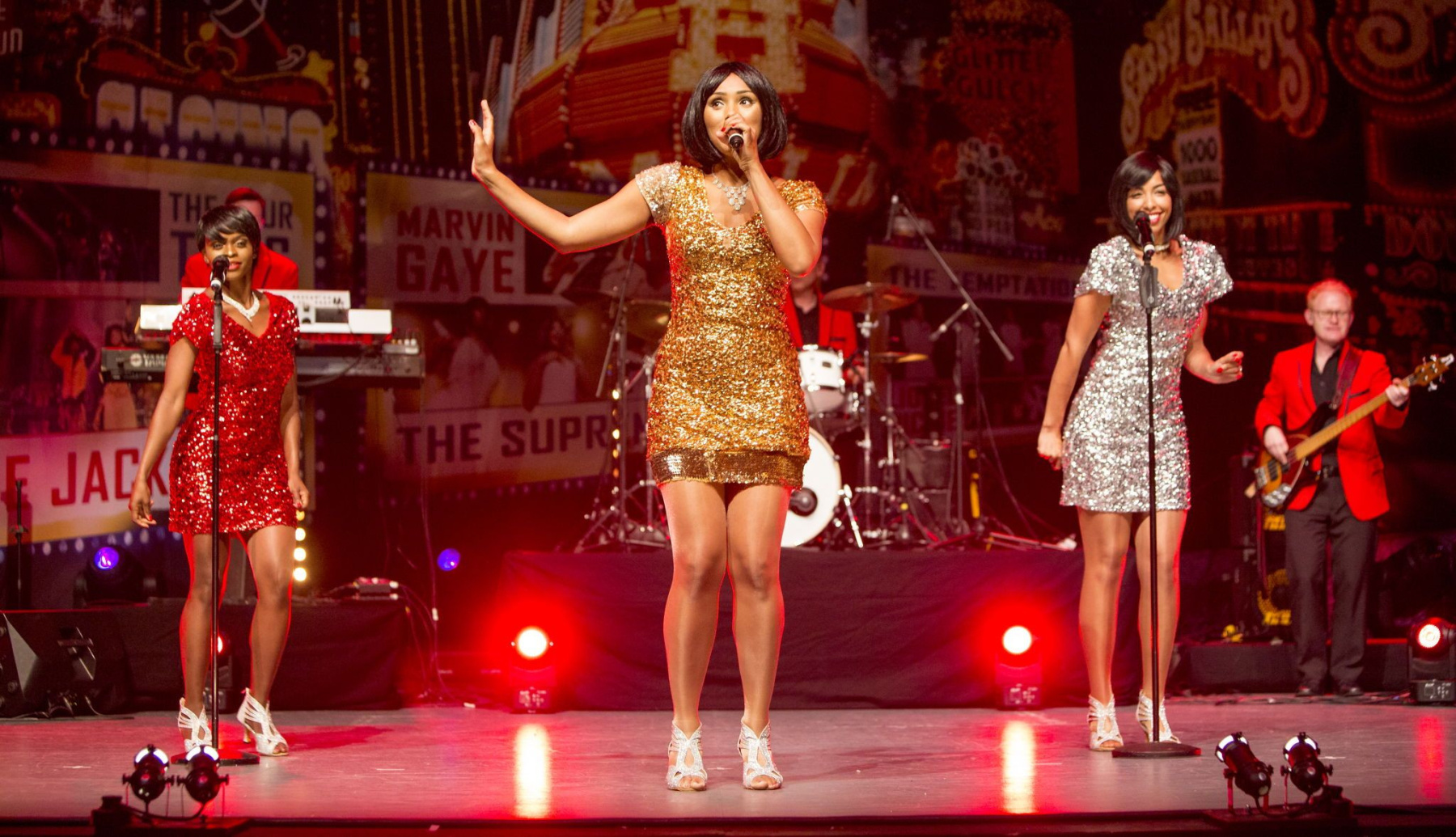The image captures a vibrant concert scene featuring three main singers and a band on stage, highlighted by the stage lights and artistic backdrop. In the foreground stands the lead singer, adorned in a dazzling, sequin-covered gold mini dress, paired with silver lace-up sandals that wrap around her ankles. She has a short black bob hairstyle and is holding a microphone close to her lips, her right arm raised slightly with the palm facing outward as she sings. To her left and right are two backup singers, each also sporting short black hairstyles. The singer on the left wears a striking red dress and a large white necklace, while the singer on the right dazzles in a sparkling silver dress; both are clad in similar lace-up sandals and appear to be dancing with bent knees and twisting hips.

The stage is occupied by a band in the background, featuring a keyboard player, a bass guitarist dressed in a black shirt, trousers, shoes, and a red coat, and a drummer partly hidden but identifiable by his white drum set and cymbals alongside a long, extended microphone. Notably, the background also displays names such as Marvin Gaye, The Supremes, and Sassy Sallies, amidst a shiny, possibly hardwood, stage floor accented by red stage lights. The musicians are dressed in red jackets, adding to the cohesive visual harmony of this energetic and dynamic concert moment.